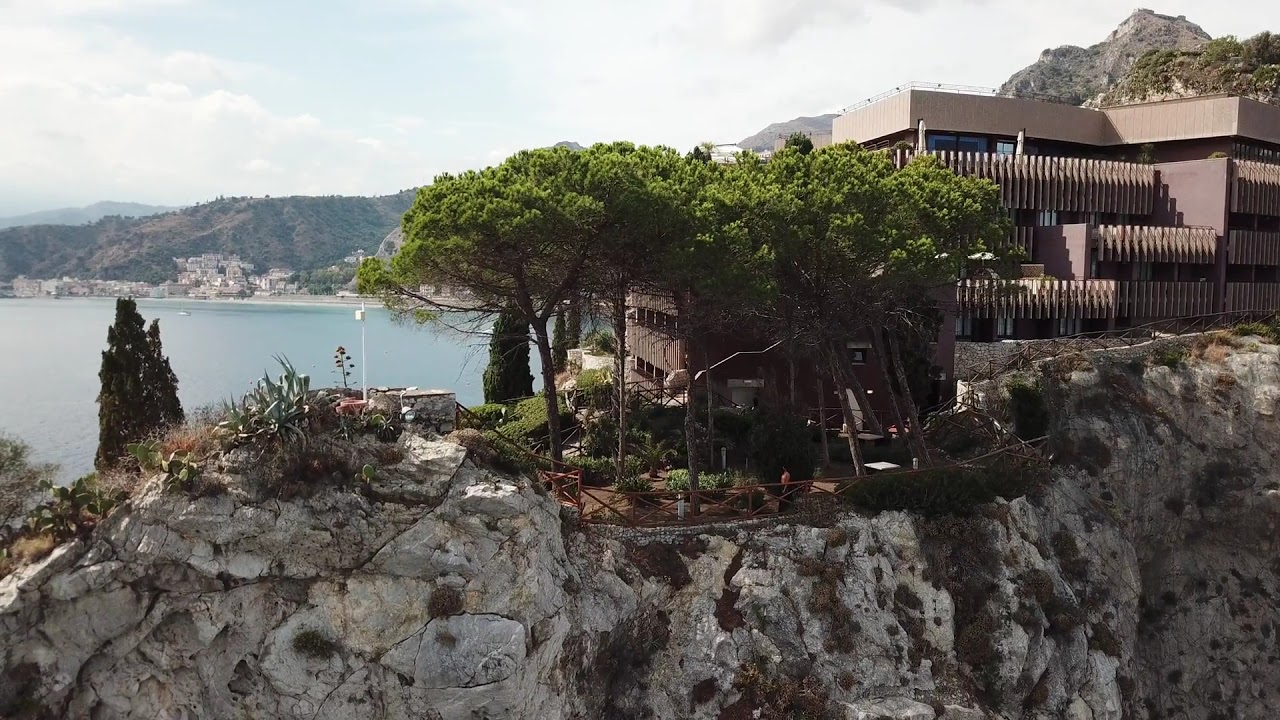The image captures a clear and detailed outdoor scene during daytime, featuring a rocky cliff or ridge jutting into a light blue body of water, likely an ocean or lake. Centered on this cliff, which extends from the bottom up to about halfway through the photograph, is a small grove of lush green trees. Situated towards the upper left of the frame is a modern, brown, terraced building, resembling a three-story concrete structure with fences near its front, possibly an office or an upscale house. This building rests on the ridge and integrates with the landscape, including a small lawn area with an antenna post on top. Further back, the ridge is flanked by more greenery and another two-story building partially obscured by trees. In the background, the hillside and partly cloudy blue sky add depth to the image. The photograph contains no humans or vehicles, emphasizing the natural and serene surroundings.